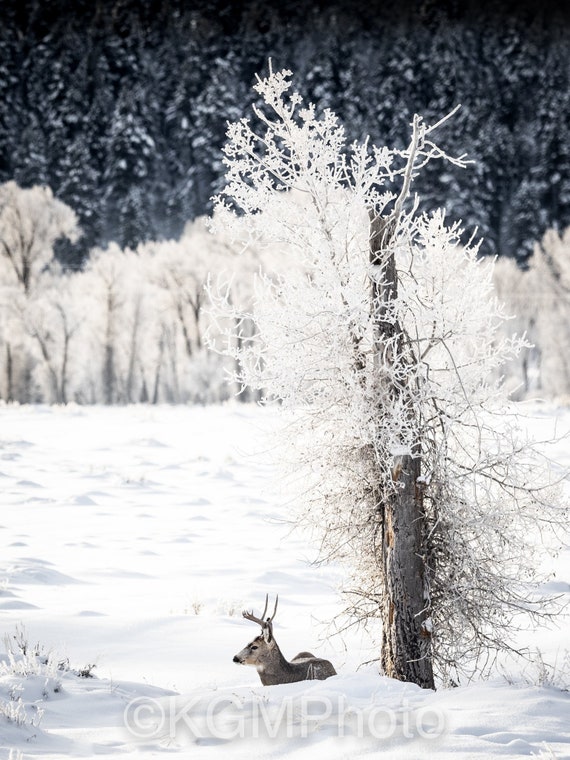The photograph captures a serene winter landscape bathed in daylight. In the foreground, a deer with antlers sits partially buried in deep snow near the base of a large, bare tree whose frost-covered branches stretch out in various directions. Surrounding the deer and tree are tall snowbanks dominating the lower portion of the scene. A line of snow-covered deciduous trees extends across the middle ground, their branches blanketed in thick snow and ice. Behind these trees, a backdrop of evergreen pine trees, dusted with snow and slightly out of focus, creates a layered depth to the image. The sun illuminates the scene, casting a soft glow over the entire snowy expanse. A watermark reading "copyright KGM photo" is visible at the bottom of the image.